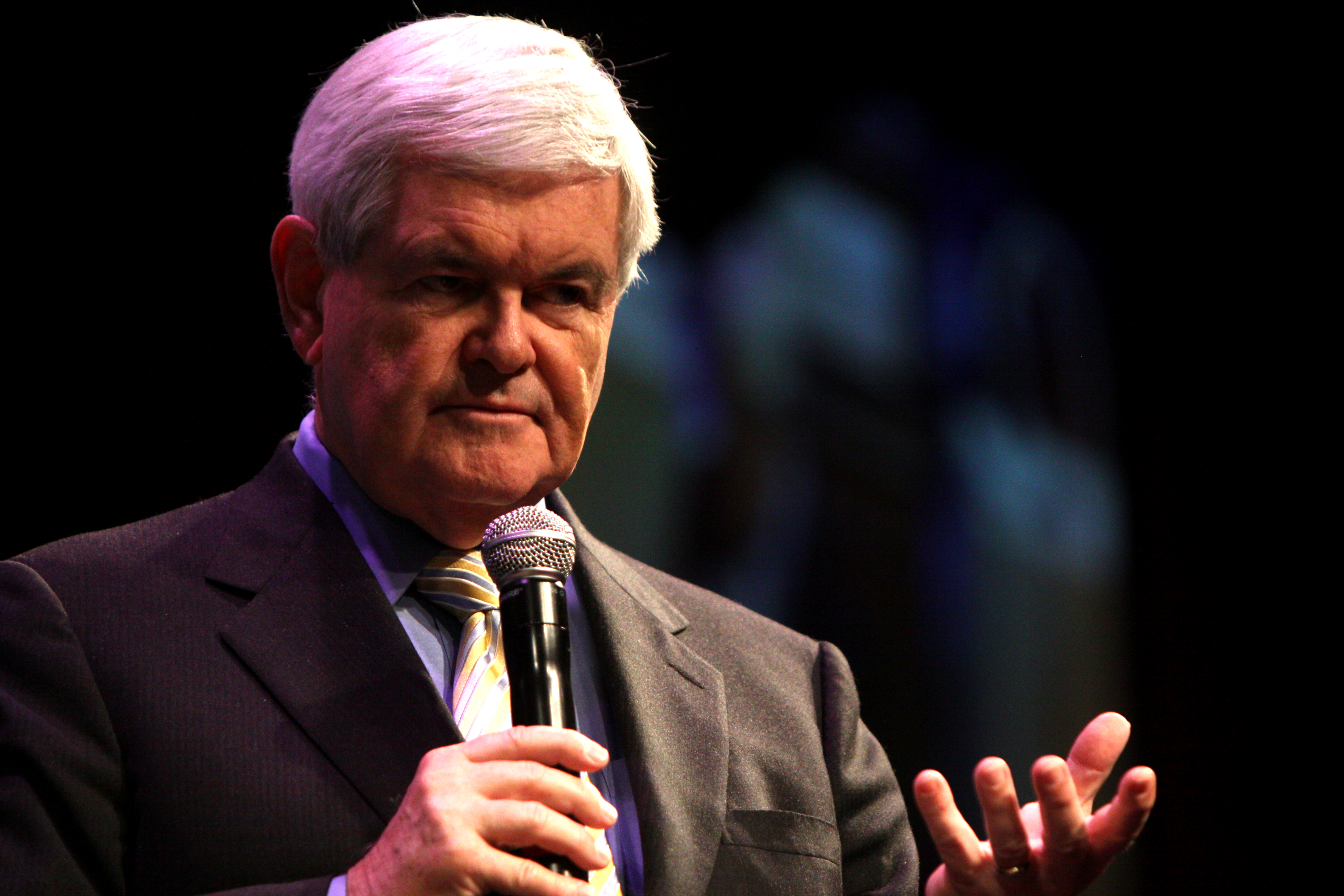In this image, the scene is set indoors in a dark, dimly lit room, likely during a speech or presentation. The background is predominantly black and relatively blurry with scattered areas of white and blue, adding to the ambiguous and indistinct ambiance. The primary focus of the image is a man positioned centrally, slightly to the left. He has thick gray hair and a serious expression as he looks off to the right, presumably addressing a crowd. He is dressed in a gray suit jacket over a blue button-down shirt, complemented by a yellow tie with diagonal blue stripes. The man is holding a microphone near his chin with his right hand, his elbow bent at more than a 90-degree angle, his palm facing upward, suggesting he is in the midst of explaining something or engaging the audience. No text is visible within the image, directing all attention to the man's poised demeanor and the subtle, yet varied color palette of black, white, tan, gray, silver, and purple.